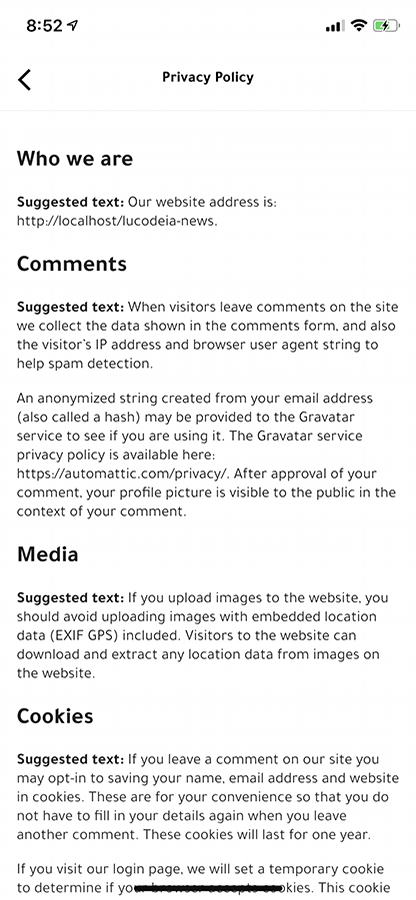Screenshot of the Privacy Policy Section in a Mobile App:

At the top left of the screenshot, the time is displayed as 8:52 and location sharing is enabled. The top right corner indicates strong connectivity with three out of four bars of mobile signal, full Wi-Fi strength, and a charging battery at 50%, denoted by a small thunderbolt icon.

The main screen shows a white background with "Privacy Policy" written in black font at the center. Below it is a solid black line separating the header from the content. The privacy policy section begins with the heading "Who we are" followed by "Suggested text:" and provides a placeholder URL: "http://localhost/LucaDiaNews".

Further down, the policy addresses "Comments" and specifies: "Suggested text: When visitors leave comments on the site, we collect the data shown in the comments form, along with the visitor's IP address and browser user agent string, to help with spam detection. An anonymized string created from your email address (also known as a hash) may be provided to the Gravatar service to check if you are using it. The Gravatar service privacy policy is available here: https://automatic.com/privacy/".